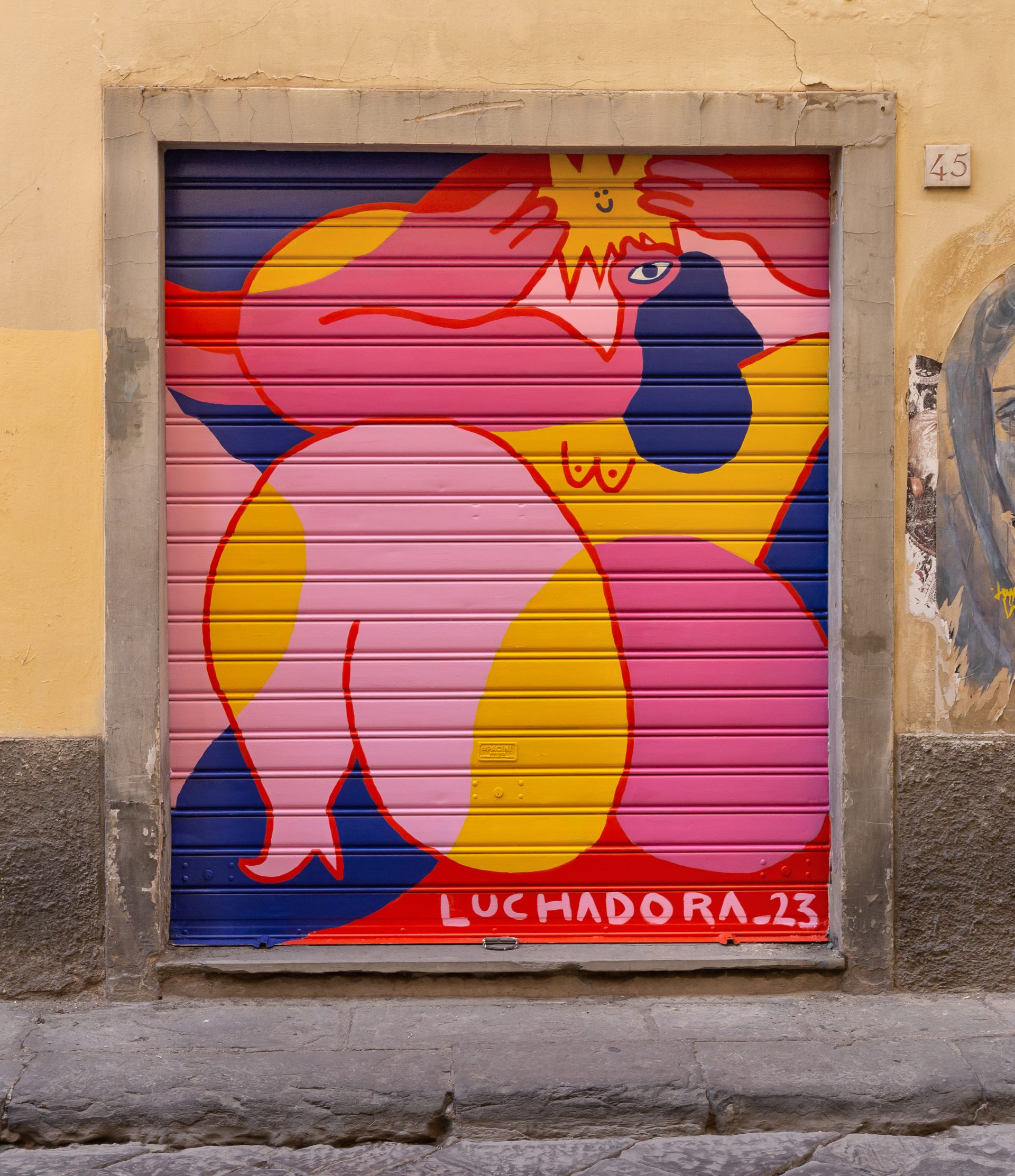The photograph captures an outdoor scene featuring a storage shed with a distinctive, custom-painted metal door framed by a weathered, beige-beige colored concrete wall. The door, which slides up into the ceiling, stands on a slightly elevated step composed of small bricks, in front of a brick-like street. This unit, labeled as unit number 45 by a small sign in the upper right corner, is adorned with an artistic mural signed "Luchadora 23" in pink letters on the bottom right.

The mural is a vibrant and bold modern art piece, dominated by bright colors—pinks, yellows, blues, and reds—and characterized by its simplistic yet striking design. Central to the artwork is a stylized figure of a woman, seemingly worshipping the sun, depicted with just one visible eye and three fingers on each hand. Overhead, a small, smiley sun smiles down on the scene, adding a playful element to the otherwise exaggerated and artistic interpretation of the figure.